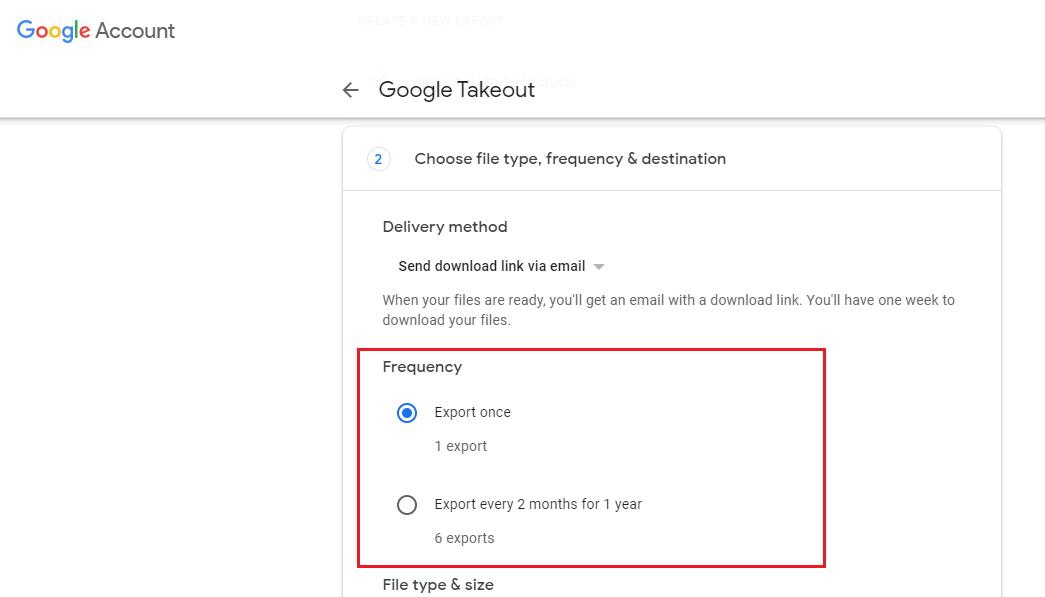**Detailed Caption:**

The image depicts a Google Account page with a clean white background. At the top left corner, the Google logo is prominently displayed next to the word "Account" written in gray. Centered in the top section of the screen, the page displays the tab title "Google Takeout" also in gray.

Below this title, in the main body of the page, there's a large white box that dominates the center of the interface. Within this box, on the top left, there is a blue number "2" encircled by a light blue circle. To the right of this circle, bold black text reads "Choose file type, frequency, and destination."

Below this header, the next section is labeled "Delivery method." The text is followed by a dropdown menu, which is currently set to "Send download link via email." This indicates the preferred method of receiving the exported files. Directly beneath this, a helpful note specifies: "When your files are ready, you'll get an email with a download link. You'll have one week to download your files."

Further down, the section labeled "Frequency:" shows two options, with the "Export once" option selected. This part of the interface is marked with an edited red box, drawing attention to this specific setting.

Clearly, the screenshot serves as a guide to illustrate the steps required to export files using Google Takeout, highlighting the selection of file type, frequency, and delivery method for the download process.